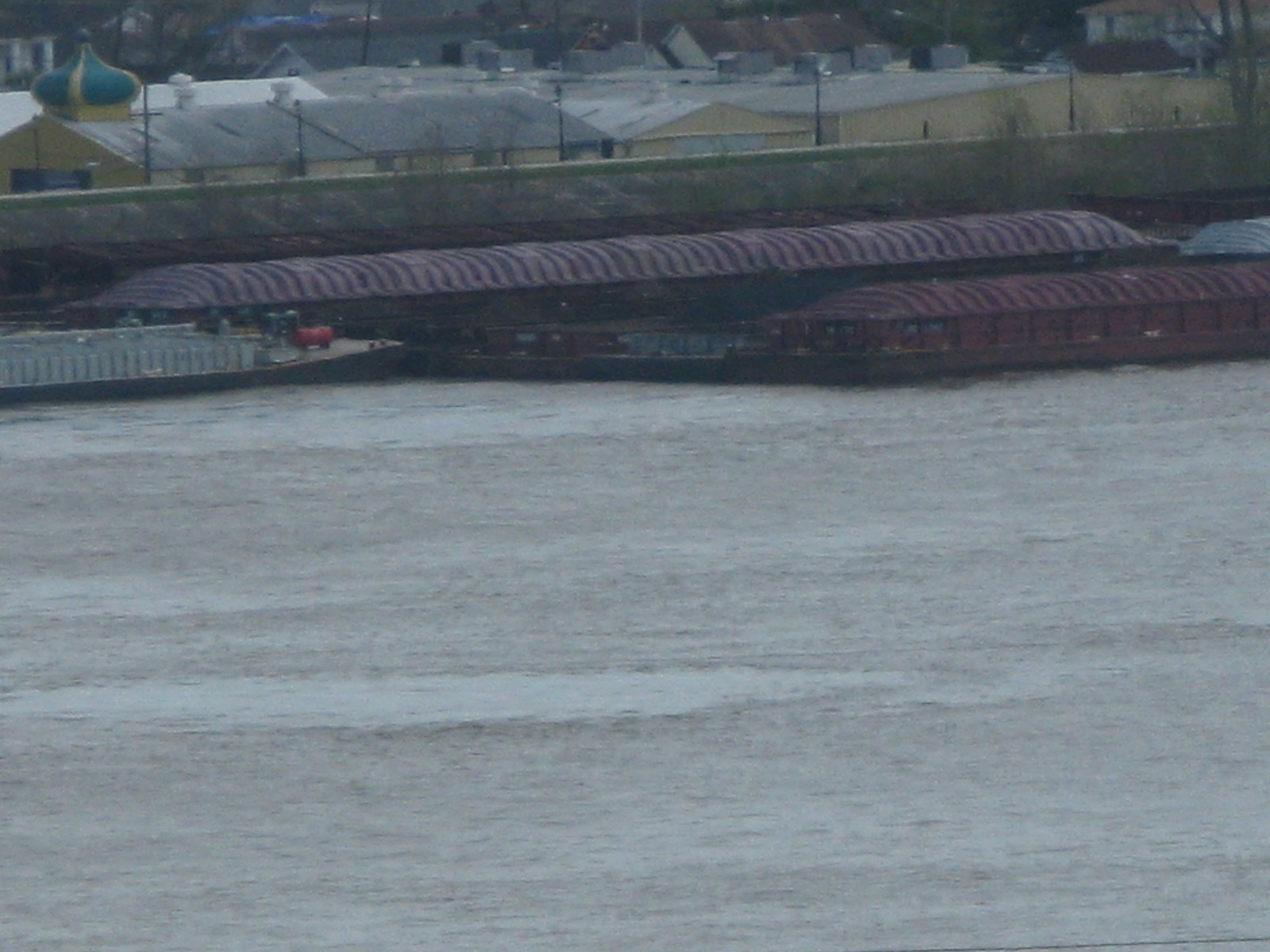The image showcases a serene body of water in the foreground, with its surface appearing exceptionally still and gray. Spanning the background is a bridge or cement wall that stretches across the length of the water, creating a barrier between the water and the cityscape beyond. Alongside this wall, several long, maroon, floating structures resemble old boats or train cars, and they appear rusted with reddish-brown rooftops and ridged designs. One of these floating structures seems to have windows, adding to their intrigue.

To the left of these structures, there is a boat with a distinctive triangular front, featuring a white railing and a red object at its tip. Additionally, a red barrel can be seen on a deck in the same area. Beyond the bridge or wall, there are single-story houses painted in light beige, each capped with gray rooftops. Among these buildings, a notable decorative dome, blue with golden accents, rises on the top left. The overall scene is tranquil, with the calm water and the mixture of historical and architectural elements painting a picturesque and detailed landscape.